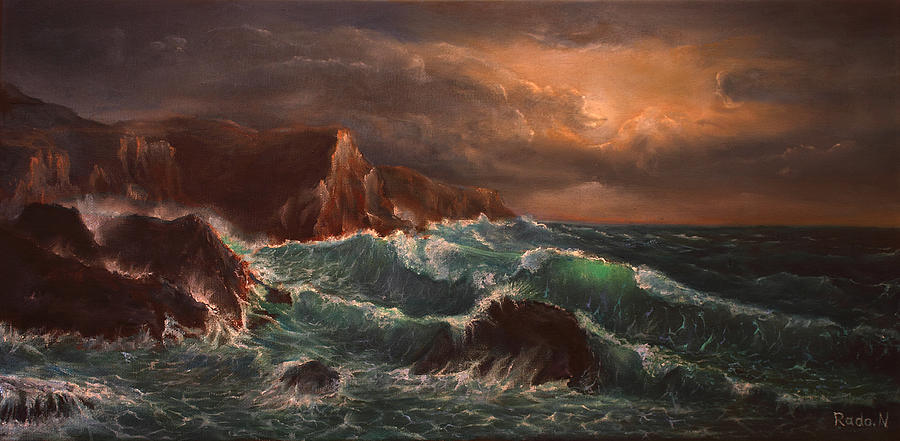This artwork is an oil painting depicting a tumultuous ocean scene. The sky is predominantly dark and stormy, with grey storm clouds enveloping the scene. However, a small portion of the sun peeks through the clouds, casting an orangish glow in the center. The ocean waves are violent, crashing against jagged, rocky cliffs on the left side of the painting, with some smaller black rocks visible at the bottom. The water transitions from a dark blue near the rocky shoreline to a lighter aquamarine green towards the center, where waves appear calmer as they approach the horizon. In the bottom right corner of the painting, there is a handwritten signature that reads "rada.n" or "Radha N," presumably the artist's name.